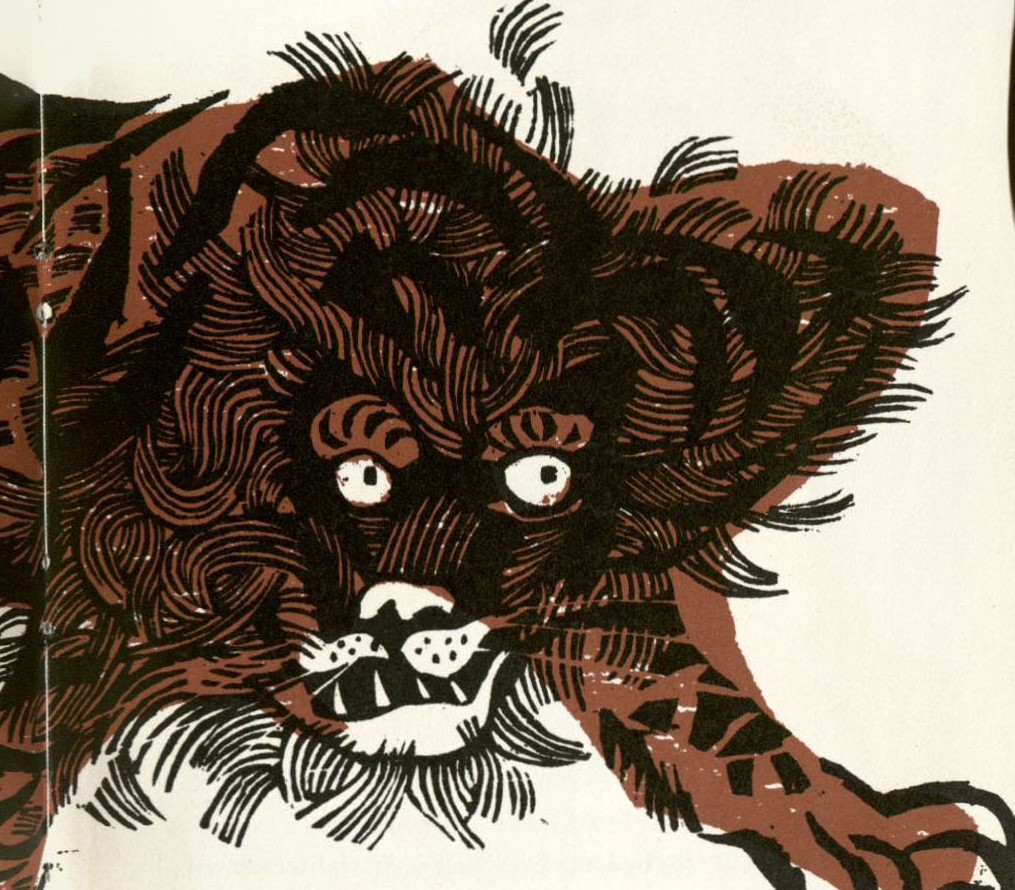The image depicts a modern interpretation of a stylized lion, resembling wood carving artwork. The illustration, set against a soft cream-colored, aged beige background, stretches within a wide vertical rectangular frame. Enhanced by a visible crease or white line on the left side, suggesting a fold or string, this gives it the look of vintage cover art, possibly for a book.

The lion’s form is defined by thick black lines, providing its mane, hair, and fierce details like around the eyes and mouth. The creature, in mid-step from the left to the center, twists its head to face the viewer. Its fur is rendered in a dark, reddish-brown color, contrasting sharply with its white eyes, teeth, nose, and claws. The eyes, with noticeable black dots that add an intense gaze, stand out prominently. While some described it as demonic or evil-looking with big pointy teeth, the overall aesthetic is a striking blend of dark brown and black on the aged background, emphasizing the intricate, almost wood-cut styled artistry of the piece.